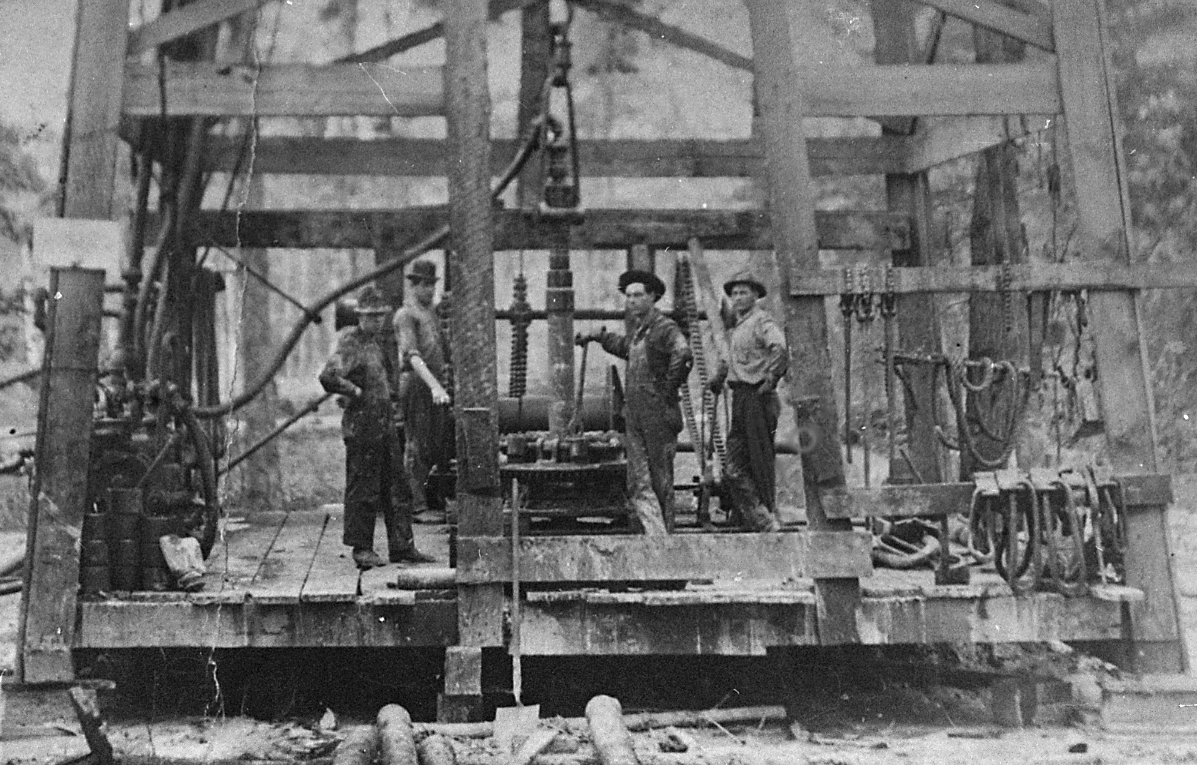A vintage black-and-white photograph captures an early 20th-century oil drilling rig, framed by a wooden structure with open sides and metal I-beam girders. In this grayscale image, four men stand on a platform made of wide wooden planks, surrounded by an assortment of industrial equipment, including pipes, cables, winches, and hoses. This setup, likely dating from the late 1800s to the 1920s, shows a hydraulic-powered drill apparatus with auger-like shapes and chain-driven mechanisms. The men, possibly worker attire from the 1910s to 1940s, are dressed in denim clothing and hats—some wearing bib overalls, others in work clothes, and one with a bowler hat. They pose around the central drill, two with hands resting on their hips, and face the camera with a serious demeanor. The backdrop hints at the challenging working conditions of an early drilling site, with messy grounds and hints of toweringly tall trees visible through the open structure.